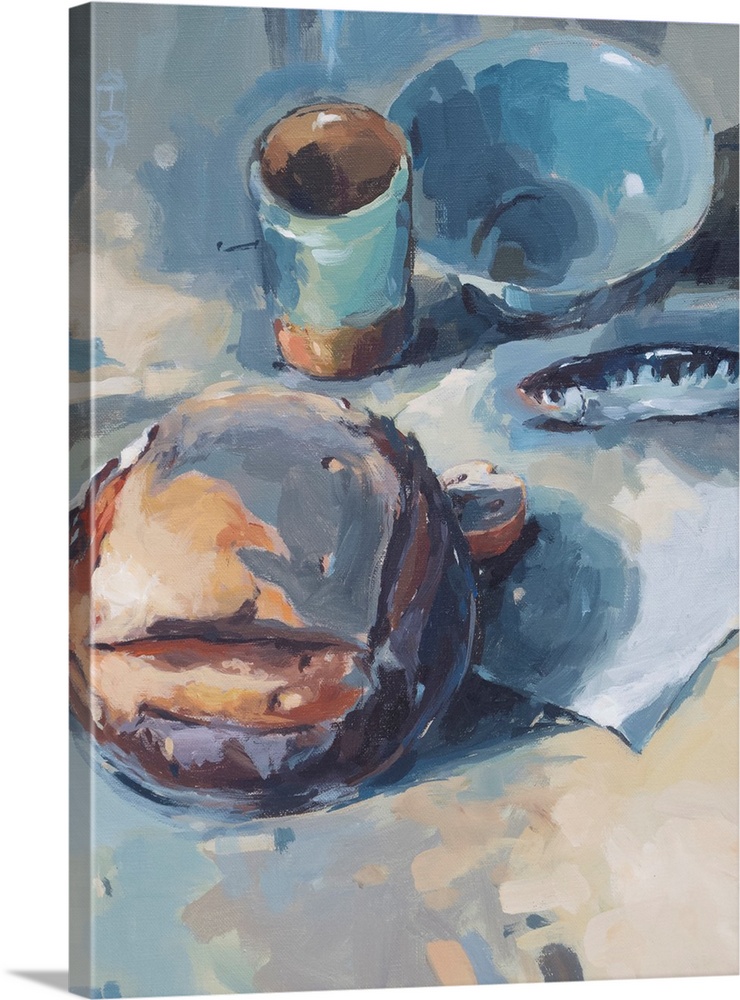This surreal painting features a blue bowl in the upper right corner, distinct with its darker and lighter blue shades blending inside. Adjacent to the bowl is a two-tone mug, brown at the bottom and blue at the top and inside, filled with a brown liquid. Below these objects lies a gray, round object with a couple of holes, transitioning to an orange hue towards the lower right. A prominent element of the sketch is a fish with a dark top, white reflective highlights, and a gray underside, positioned on a white piece of paper that has a square in the bottom right corner and a jagged top edge. The painting's background and surface are a chaotic mix of light brown, gray, and light blue hues. The overall paint application is sporadic and lacks clarity, creating an abstract impression. Additionally, an ambiguous blue and tan object, possibly a sliced apple showing its seeds or a loaf of bread with a blue crust, adds to the enigmatic composition. The scene rests on what appears to be a blue and tan table, with a napkin casually placed atop it, against a similarly colored wall.